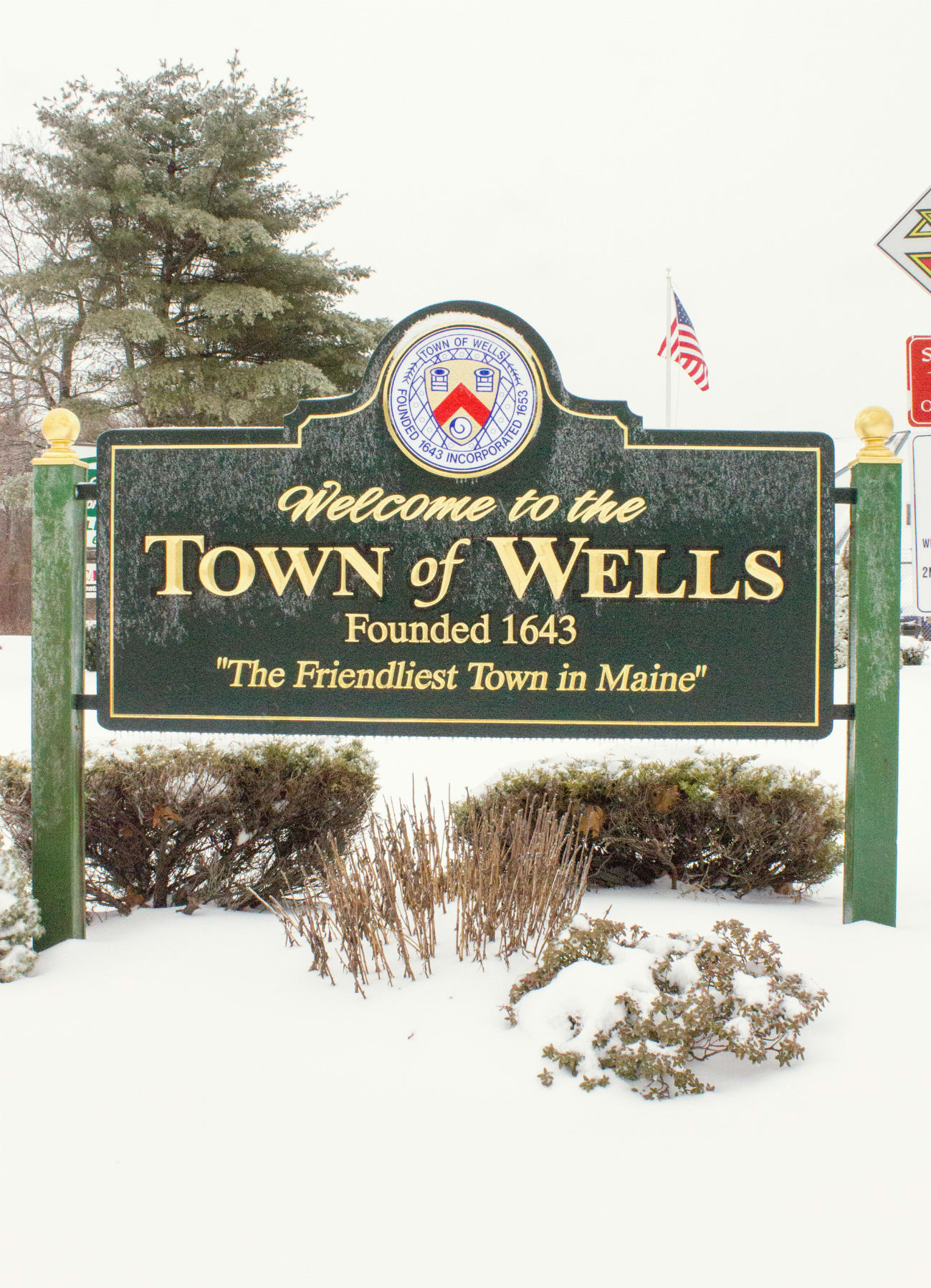In a snowy landscape, a dark green welcome sign proudly introduces the town of Wells, founded in 1643 and known as "the friendliest town in Maine." The sign, featuring light yellow font and a matching border, is held up by two identical green posts topped with gold-painted globes. At the top of the sign, a circular emblem includes the text "Town of Wells," along with "Founded 1643, Incorporated 1653" in blue and red accents. Snow covers the ground and partially buries some brown, leafless vegetation. In the background, an American flag flies from a pole, and several other signs, partially obscured, hint at additional local information.